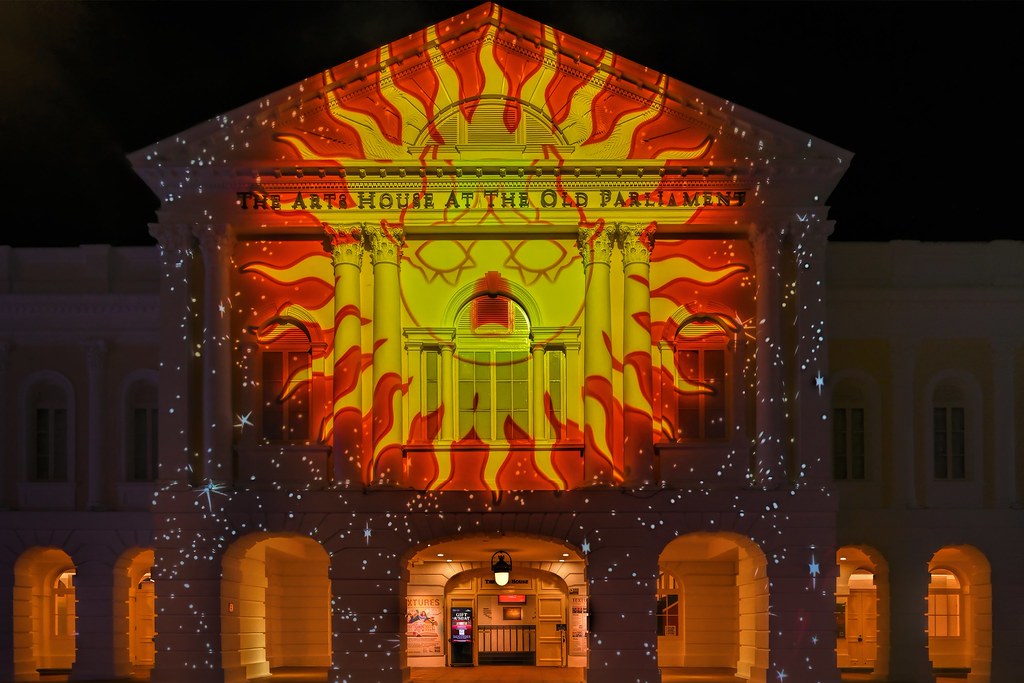This is a captivating color photograph taken at night, featuring the Art House of the Old Parliament. The image is square and concentrates on the building's detailed facade, which resembles a classic federal government style with Greek elements, including stone pillars and arched doorways. The building itself is multi-story, with a high pointed top, and its bottom row consists of several archways illuminated with a warm orange light. The largest archway in the middle prominently displays an overhead light. 

What sets this image apart is a striking projection on the building, depicting a highly detailed sun with a face. The sun's glowing eyes emit flames featuring a mix of yellow and red tones, contributing to the vividness of the projection. Surrounding the sun are red rays and sparkling white stars, creating an enthralling effect. The words "The Art House at Old Parliament" are stenciled across the top of the building, emphasizing its identity. The night sky forms a dark backdrop, making the overall scene visually dramatic and stunning.